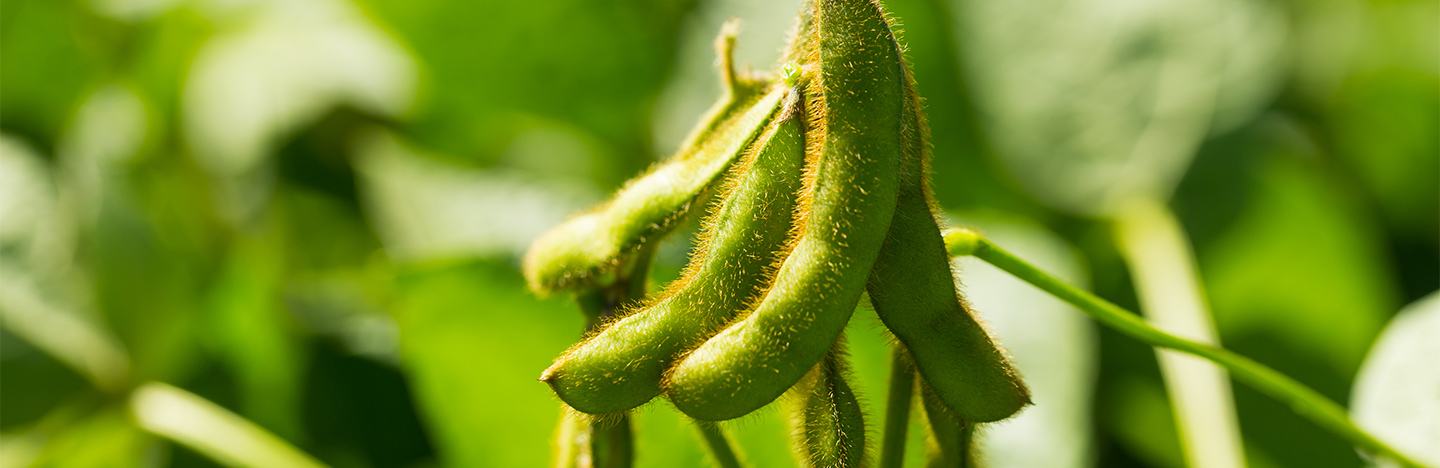This thin rectangular photograph captures a cluster of four or five fuzzy, plump seed pods that resemble pea pods. Bathed in sunlight from the upper left-hand side, the fuzzy surface of the seed pods glistens with a faint yellow glow. These seed pods are attached to a green stem, and although the background is blurred, it hints at various green shapes of additional foliage and plants, suggesting the photo was taken in a garden or peapod field. The clear daylight conditions further enhance the natural beauty of the scene, focusing the viewer's attention on the intricately detailed seed pods.